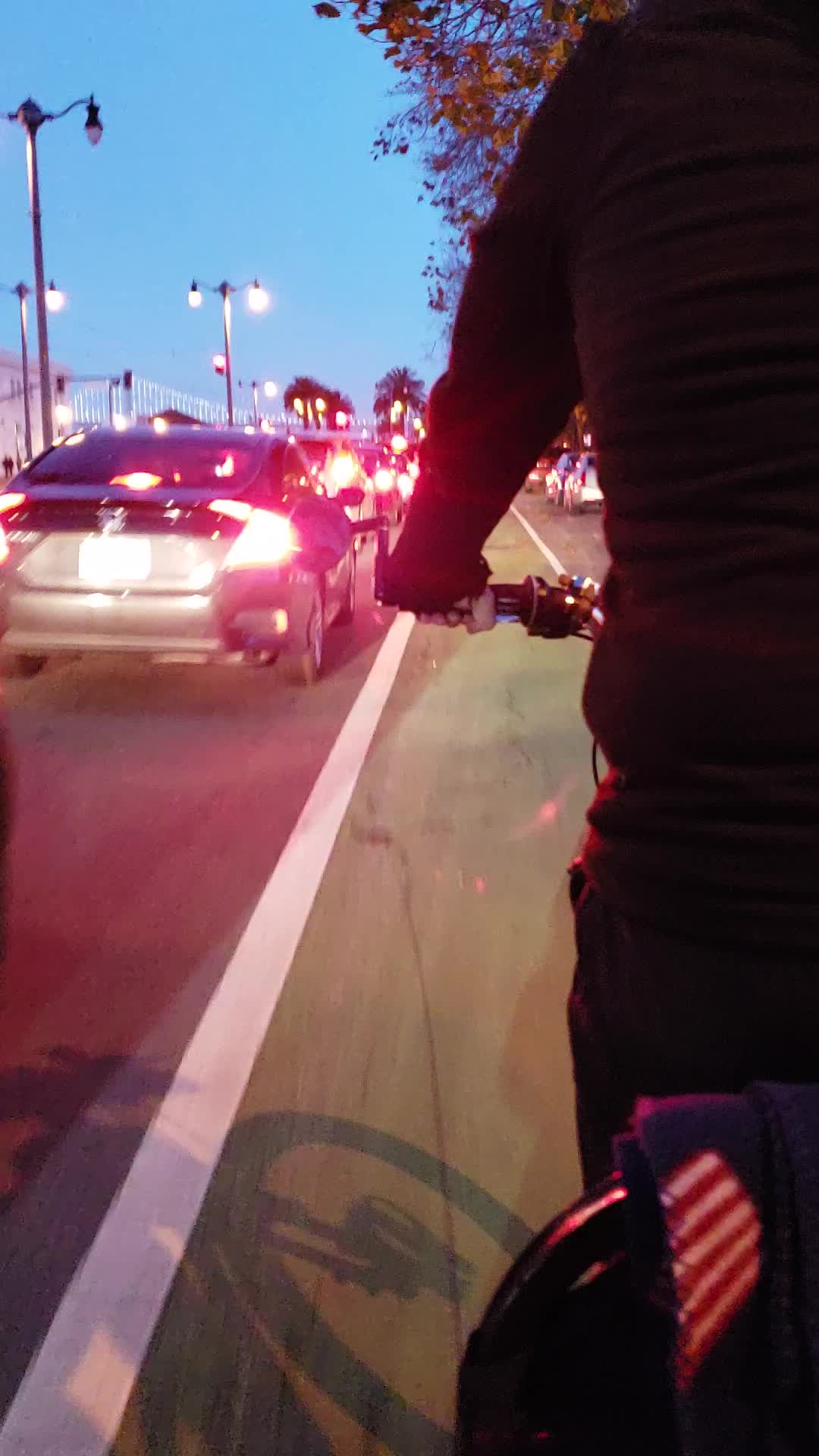This color photograph, captured at dusk, showcases a street scene with a bike lane. The viewer's perspective is directly behind a cyclist dressed in dark attire, riding down the lane. To the left, a row of cars with illuminated brake lights, led by a silver sedan, are lined up along the black asphalt roadway with white lane markings. The sky, a gradient of deepening blue, is visible in the upper left corner, complemented by street lamps and fencing. Palomino trees populate the distant background, adding a touch of greenery. The cyclist's left arm, shoulder, back, and leg are clearly visible, as is their bike's shadow extending to the bottom left of the frame. Scattered trees with full leaves are present in the upper right, enriching the scene with natural elements.